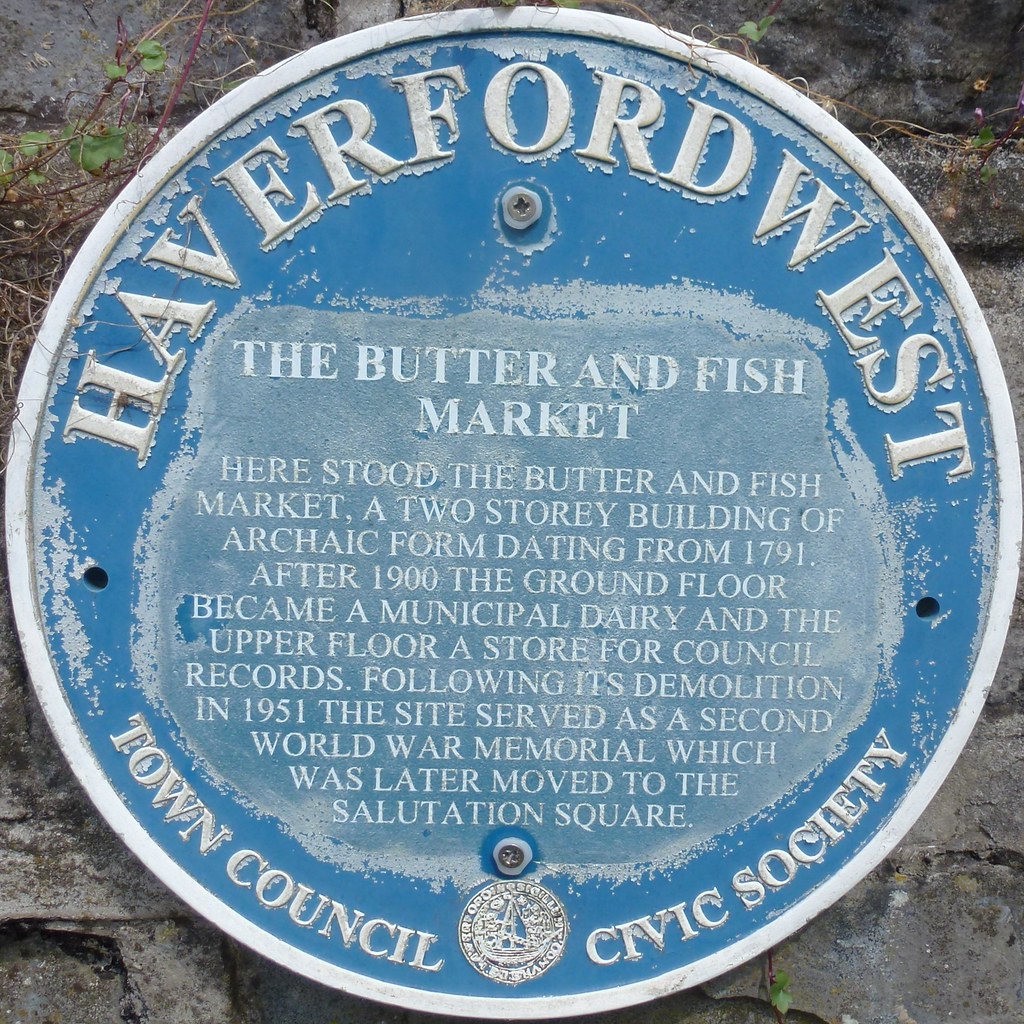The image features an old, circular, metallic signboard with a blue, rusting, and peeling finish, hanging on a dark gray stone wall adorned with vines and surrounded by bushes and rocks. The sign’s text, predominantly in white and silver, is in all capital letters and styled in Times New Roman font, with the major headings in a larger font size. At the top, curved around the sign's edge, it reads "HAVERFORD WEST." Inside the circle, the text continues with "THE BUTTER AND FISH MARKET." The full inscription commemorates the site of the Butter and Fish Market, a two-story building dating back to 1791. It notes that after 1900, the ground floor was converted to a municipal dairy, and the upper floor stored council records. It also mentions the building's demolition in 1951 and its subsequent role as a Second World War memorial, later moved to Salutation Square. The bottom of the sign features a logo, likely depicting a boat, flanked by the words "TOWN COUNCIL" on the left and "CIVIC SOCIETY" on the right, in a semicircular arrangement. The screws holding the sign in place are visible, contributing to the sign's aged and historic appearance.